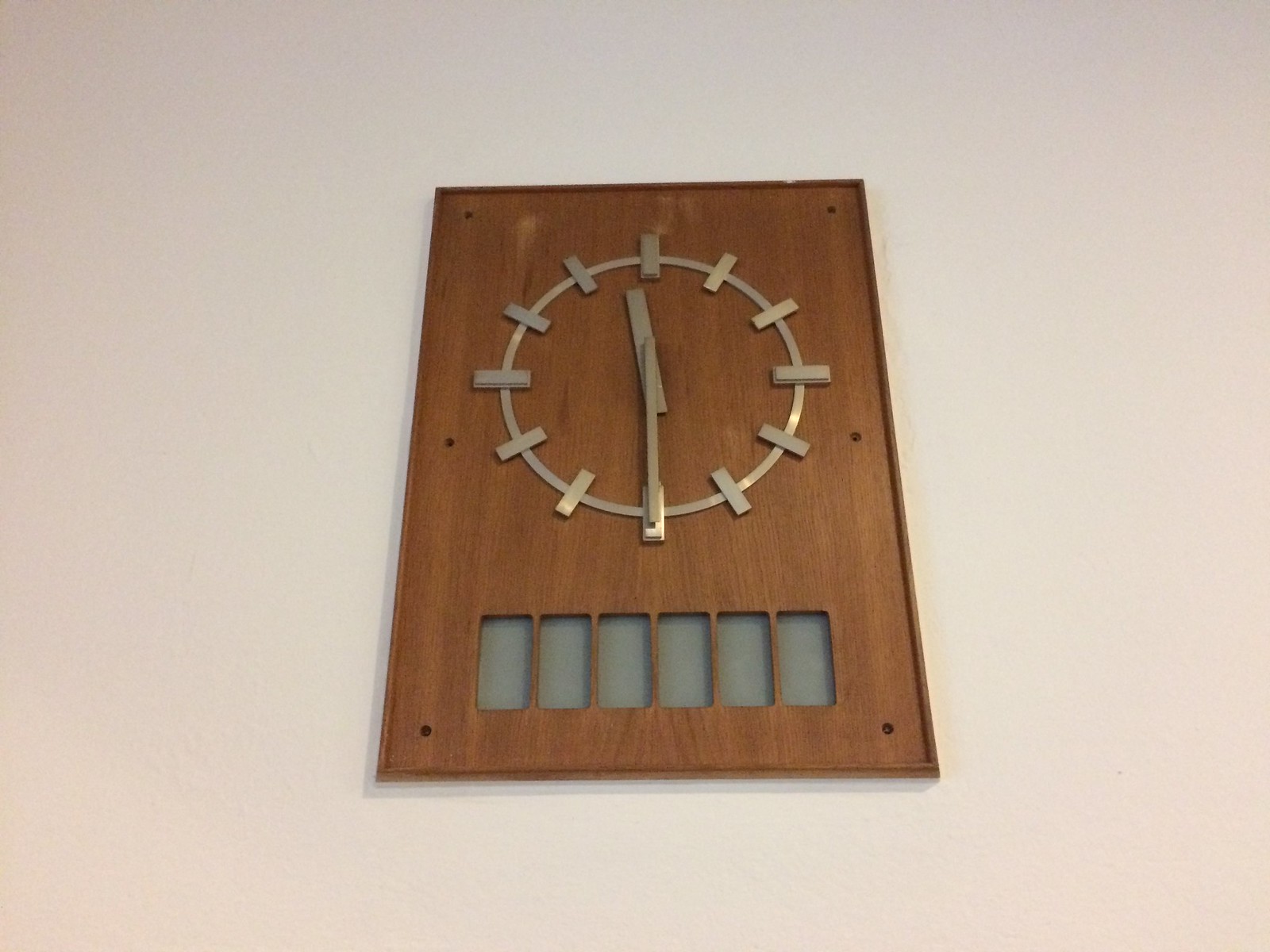A sophisticated wooden clock is mounted against a backdrop of varying shades of gray and beige. The clock features a sleek design with three screws securing each side. The face of the clock stands out as a gold circle, with gold rectangular markers indicating the hours from 1 through 12. The minute and hour hands are also gold, showing the time as 11:30. At the base of the clock, there are six vertical gray rectangles, possibly indicating the presence of a pendulum, although the pendulum itself is not visible. The overall appearance is elegant and minimalistic, blending natural wood tones with metallic accents.